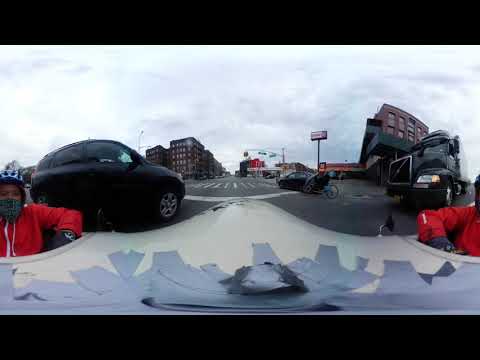This panorama photograph captures a street scene on a cloudy day, where roads, vehicles, and buildings converge into a continuous loop, taken at street level, possibly from a dash cam or a selfie stick. In the foreground to the left, a person dressed in winter clothing, including a red hoodie, green face mask, and blue helmet, appears partially submerged in a hole in the street. Surrounding this individual, a black SUV approaches from the left, while a large Mack truck with a black cabin and white trailer moves from the right. The roadway intersects with a crosswalk painted white on the dark concrete surface. The far distance reveals several tall brick buildings adorned with windows, complemented by street signs, a billboard, and various other buildings, while puffy, thick clouds loom overhead. Additional vehicles, including a bicycle, are scattered across the scene, with many more visible further back, enhancing the busy urban atmosphere.